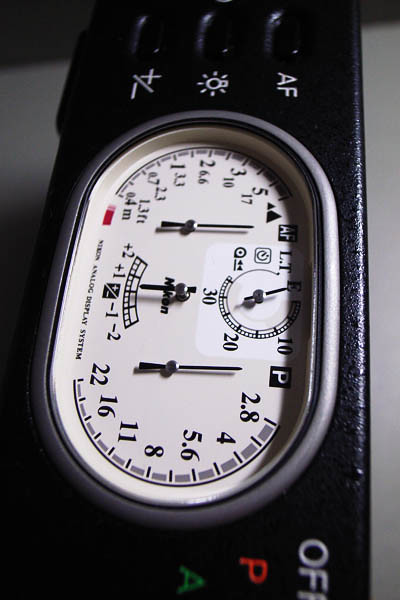This is a high-resolution color photograph of a black electronic device, prominently featuring controls and detailed markings. 

On the far left side of the device are three vertically aligned, oblong-shaped buttons. Each button is labeled with "AF" to the right. The middle button stands out with a light bulb icon that is illuminated, indicated by radiating short lines around the bulb. The bottom button is labeled with a plus-minus symbol.

To the right of the buttons, partially obscured lettering is visible. In white, the word "OFF" is clearly legible. Directly beneath this, a red letter "P" can be seen, followed by a red letter "A" below it.

The central feature of the device is a white, oblong-shaped dial encased by a silver rim. The dial is adorned with several hands of different lengths. Below this dial, the text "Nikon Analog Display System" is printed, though the exact nature of the device remains ambiguous.

On the far left of the dial, there are numeric indicators: 5, 3, 2, 1, 0.7, and 0.4. On the opposite side (far right), the numbers 2.8, 4, 5.6, 8, 11, 16, and 22 are listed, possibly indicating some form of measurement or setting scale.

The photograph captures intricate details of the device, although its precise function remains unclear.